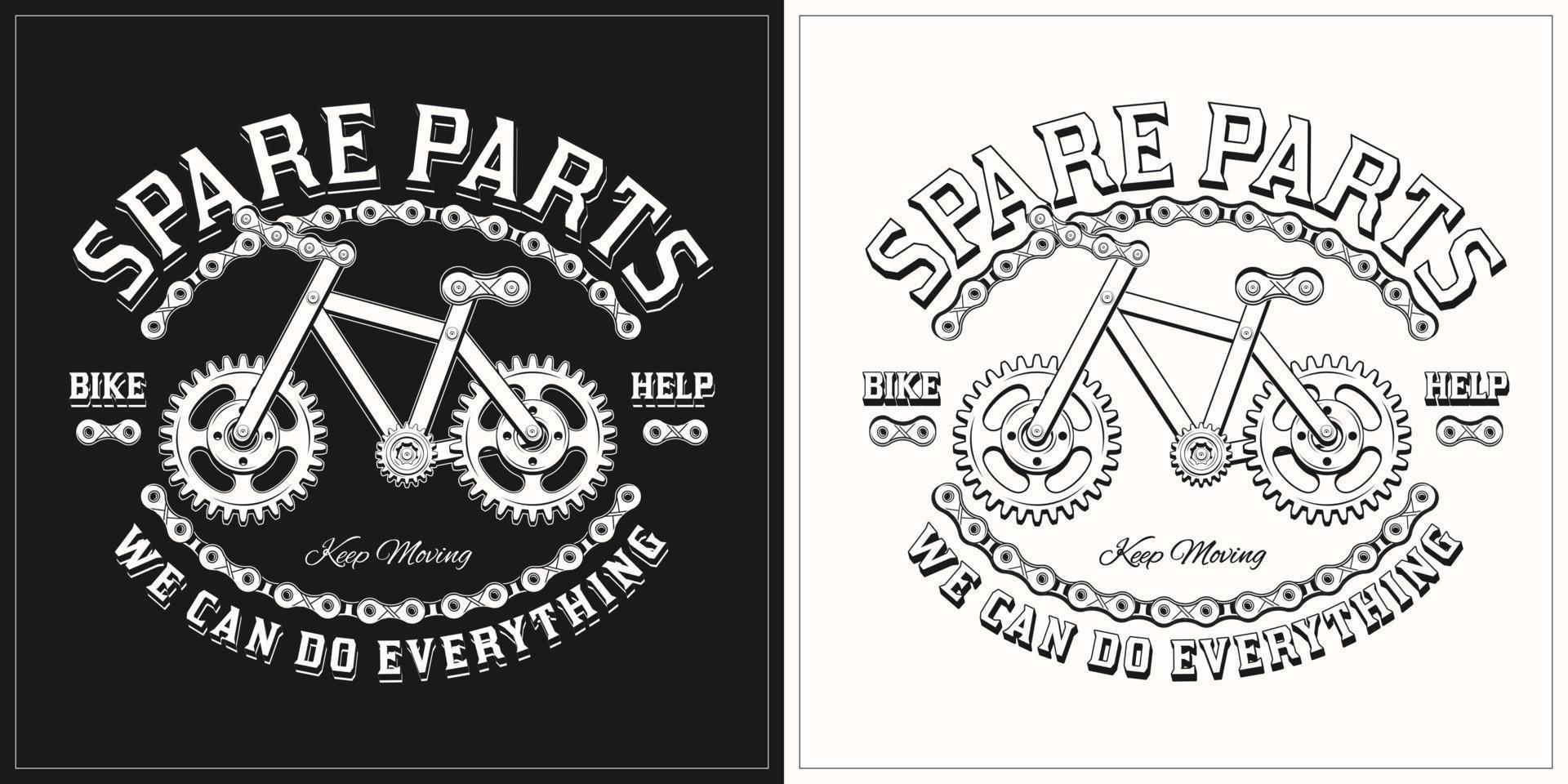This black-and-white poster is divided into two identical squares, one with a black background and white lettering and the other with a white background and black lettering. Across the top of both squares, in capital letters, it reads "SPARE PARTS," underlined by a semicircle of a bicycle chain that arcs from left to right. Below this, an intricate image of a bicycle is constructed entirely from bicycle parts and gears: the seat is made of two chain links, the tires and pedal area are represented by gears, and the handlebars are formed by a section of the chain. On the left side of the image, it says "BIKE," underlined by a small piece of the chain, and on the right side, it says "HELP," similarly underlined. Beneath the bike illustration, the phrase "KEEP MOVING" is written in cursive. Completing the design, another arch of the bicycle chain curves in the opposite direction, and below it, in bold capital letters, it states, "WE CAN DO EVERYTHING." 

The design elements are mirrored between the two squares, with the black and white colors inverted, creating a stark, visually striking contrast that maintains the same detailed, clipart-like appearance.